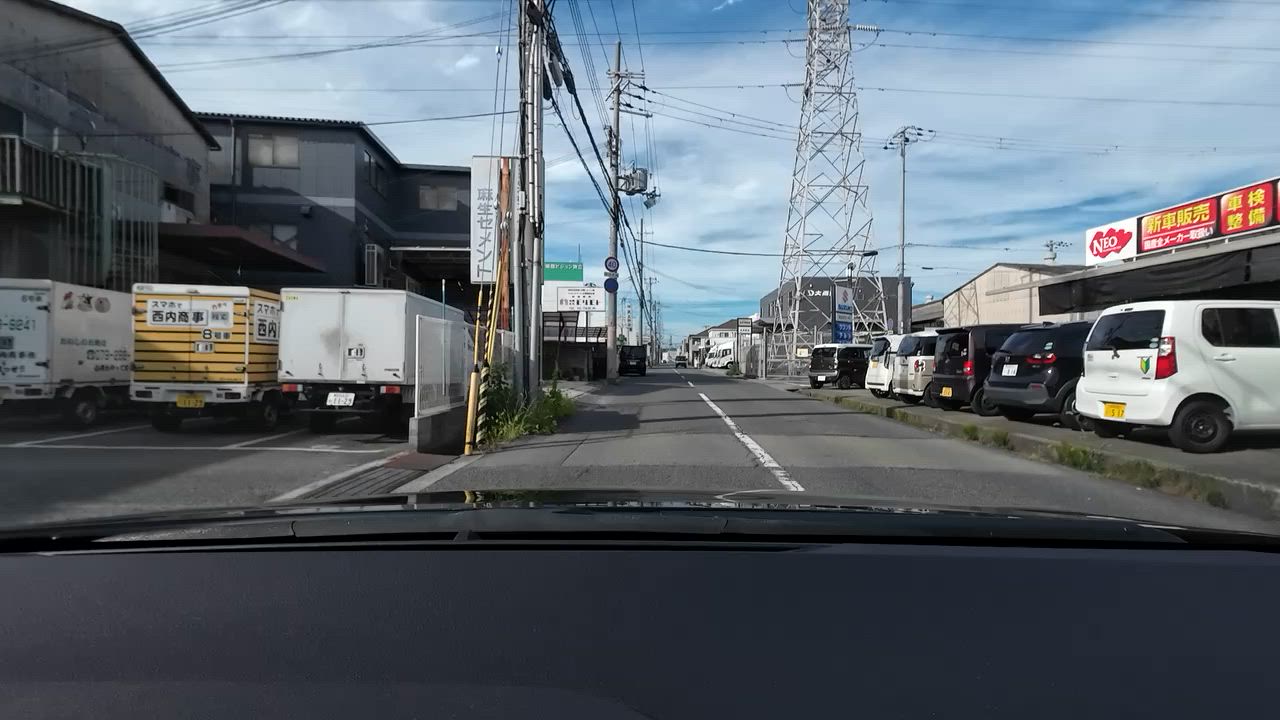In this urban street scene, a towering electric pole looms prominently in the background, flanked by numerous electrical boards and a series of poles and streetlights that line the narrow roadway. On the left side of the street, a cluster of gray apartment buildings stands adjacent to a fenced area, within which a yellow truck and a white truck are parked. The right side features a couple of businesses, identifiable by their signage — one with white and red lettering, and another with red and yellow text. A large warehouse building sits next to these businesses, with three white cars and two black cars parked in front. Further down the street, additional buildings continue the bustling urban landscape.